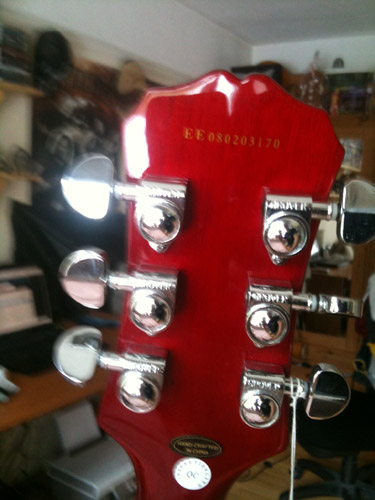The image features a close-up of the headstock of a shiny, red guitar, prominently displaying its metal tuning pegs. The guitar headstock is centered in the photograph, with the alphanumeric code "EE080203170" clearly visible on its face. Surrounding this focal point are several small, silver gauges, and a meter at the bottom with a white background containing numbers in a circular pattern.

The background of the image is blurred, showing indistinct objects that suggest it was taken indoors, possibly in a room that functions as a garage or a bedroom. The blurred background includes white walls, shelves on two different walls, a white ceiling, a brown table or desk with something silver or gray underneath, and what appears to be a printer on the floor. The colors present in the image include white, black, red, silver, brown, and gray, consistent with common household items. Overall, the scene captures a meticulous, detailed look at the guitar headstock against a backdrop of everyday residential furnishings.